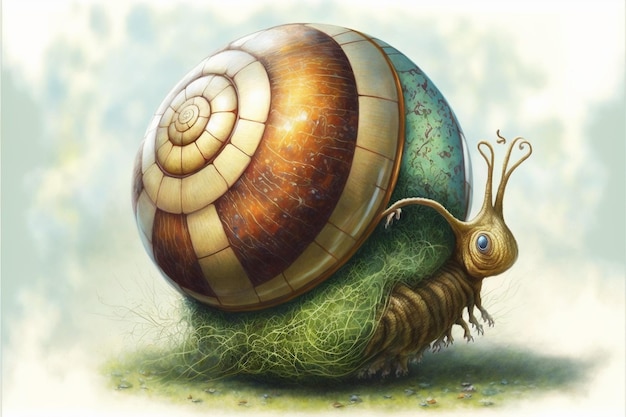This is a digitally or AI-generated graphic artwork depicting a fantasy-type cartoon snail. The snail features a large, circular shell with a detailed spiral design, including a shiny tan outer edge followed by a brown ring, and several light tan circular rings that grow smaller towards the center. The shell also has a greenish tint with brown specks and some tile-like spots, as well as a bluish hue on one side. Atop the snail's body, which is a light brown or tan color, are three or four antennas extending upwards and a blue eye looking towards the viewer. The snail's body is adorned with grass-like stringy substances and multitude of centipede-like rows of legs on both sides. It is set on a circular patch of grass in varying shades of light and dark green, complemented by dried-up brown and blue leaves. The background is a blurred, watercolor-like mixture of gray and yellow, creating a shadowy and cloudy ambiance.